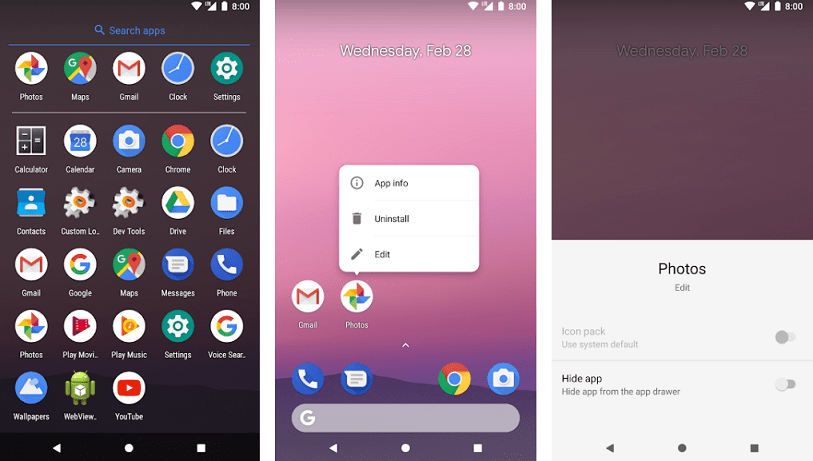This image comprises two horizontal cell phone screenshots aligned side by side. The first screenshot displays the "Search Apps" screen, revealing a comprehensive view of several app icons. At the top, there's a search bar, beneath which the "Photos," "Maps," "Gmail," "Clock," and "Settings" apps are visible. Following this, a vertical list of apps is presented including "Calculator," "Calendar," "Camera," "Chrome," "Clock," "Contacts," "Custom Dev Tools," "Drive," "Files," "Gmail," "Google Maps," "Messages," and the "Phone" app icons. Subsequently, the apps "Photos," "Play Movies," "Play Music," "Settings," "Voice Search," "Wallpapers," "View," and "YouTube" are shown. 

The middle screenshot is purely a wallpaper without any visible app icons or interactive elements, offering a serene visual contrast to the densely packed first screen.

The third and rightmost screenshot is set on the "Photos Edit" tab. This indicates that the user is in the process of editing a photo within the "Photos" app. Notably, the time displayed across all three screenshots is consistently set at eight o'clock, suggesting a synchronized capture likely done simultaneously.